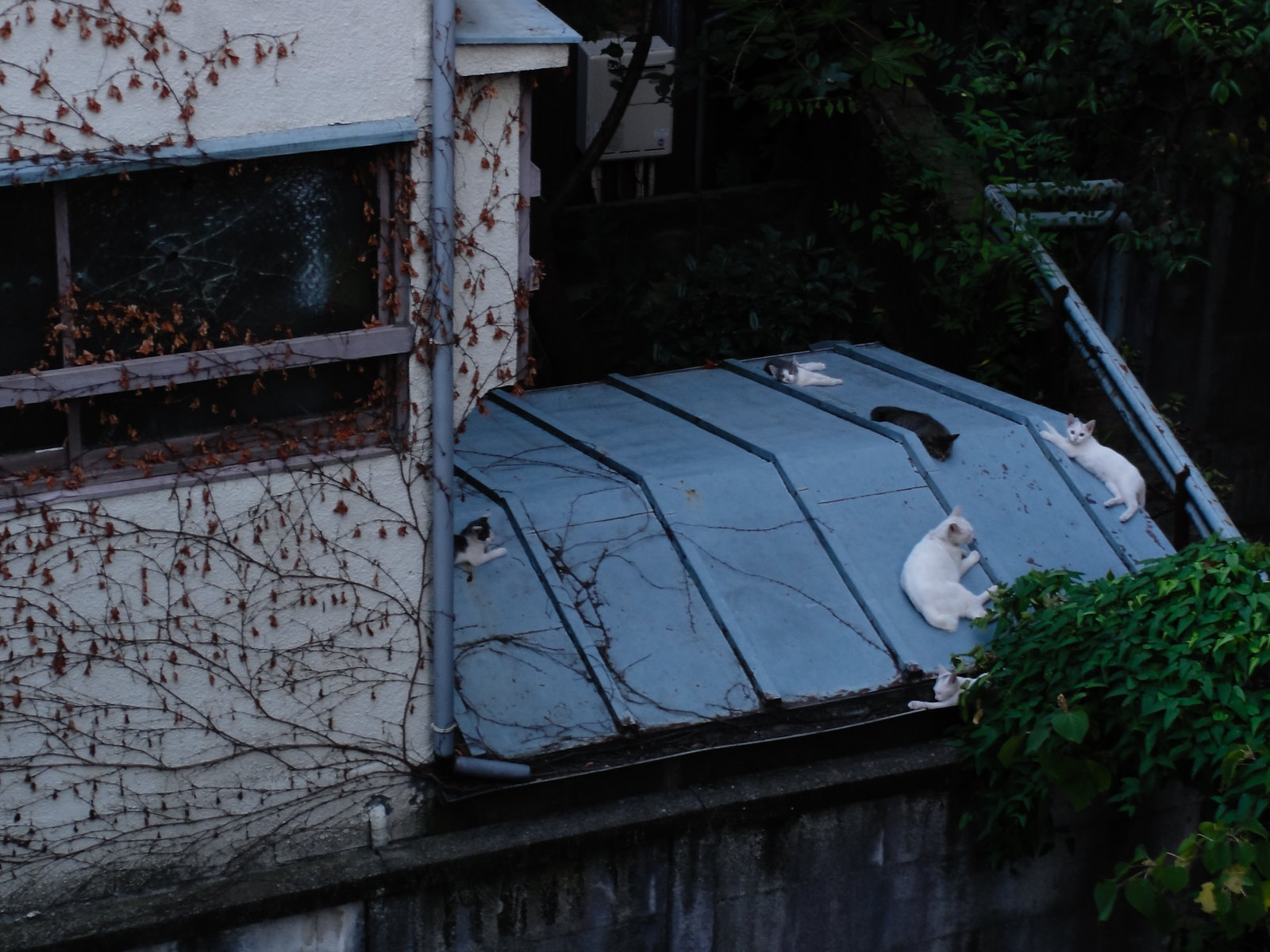The photograph captures a gloomy, overcast day, looking down from one rooftop to a blue metal rooftop across an alley. The scene is set atop a weathered white stucco building, which features light blue wooden frame windows and a barely open window with panels in light blue. Mottled with brown vines and ivy crawling up its facade, the building appears somewhat neglected. A blue gutter pipe traverses the wall, running parallel to the composition. Scattered across the roof are six cats in various states of repose: two black and white cats, one black cat, and three white cats. One cat lounges in the low-sloped gutter while others stretch across the flat sections of the roof, seemingly indifferent to the cold, damp weather. In the corner of the image, green foliage and a sizable electrical box are visible, adding to the slightly dilapidated feel of the scene.